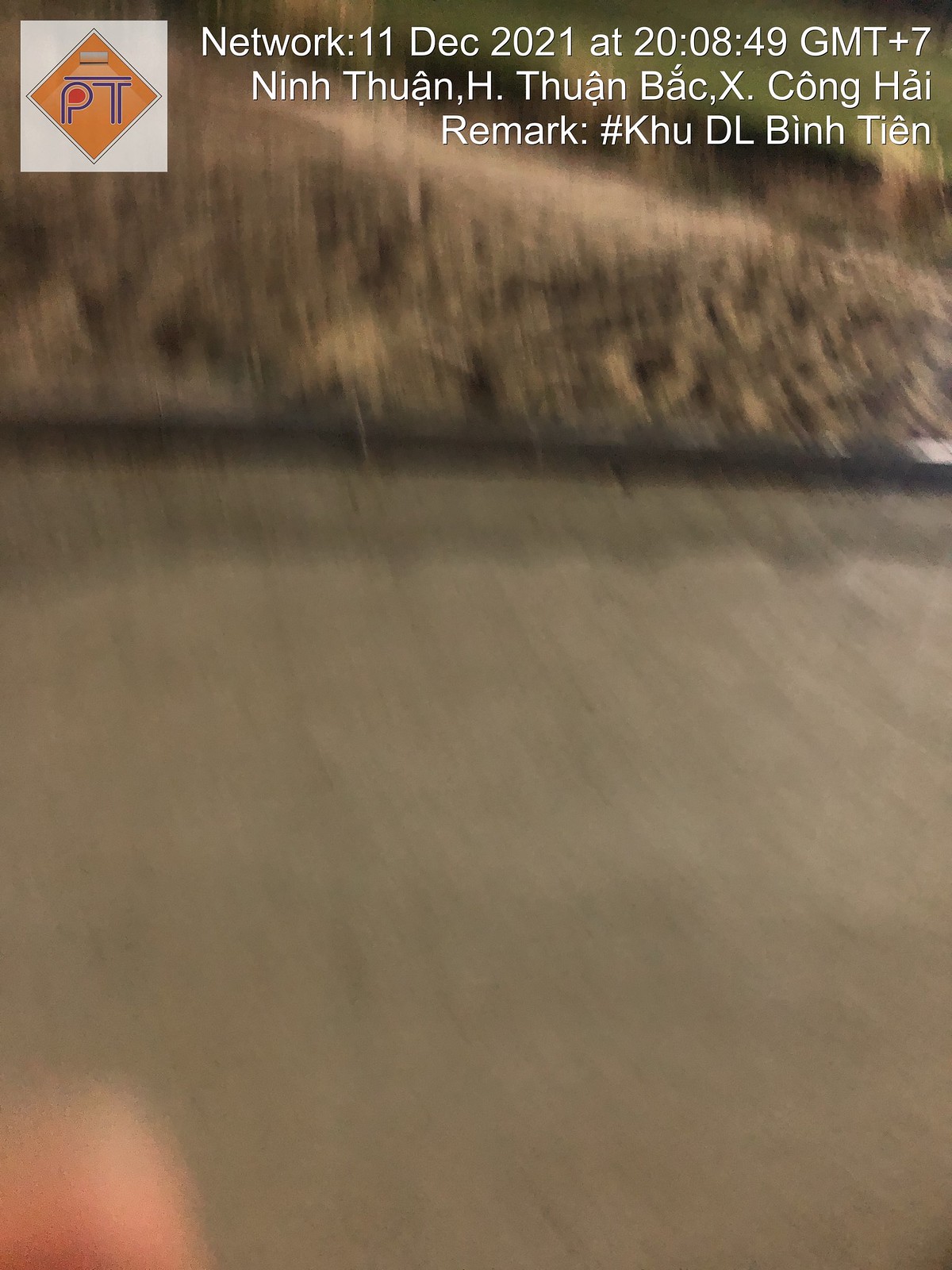This is an out-of-focus photograph characterized by a predominantly brown and tan color palette. The image features text at the top center and a logo in the upper left corner. The logo is square-shaped with a yellow-orange diamond and blue lines resembling the letters "P" and "T." Adjacent to the logo is white text displaying a time and date in a non-English script, possibly Thai.

The composition of the photo suggests a landscape scene. The lower two-thirds of the image displays a smooth, lighter tan area, while the top third depicts a darker, more textured region. This upper portion appears to rise, resembling a hill with potential shrubs or brush scattered across it. Additionally, in the lower left-hand corner, there is a peach-colored circle, possibly a person's hand, partially visible.

Overall, the photo’s lack of clarity makes it challenging to discern precise details, but the combination of the elements provides a hint of a natural outdoor setting.